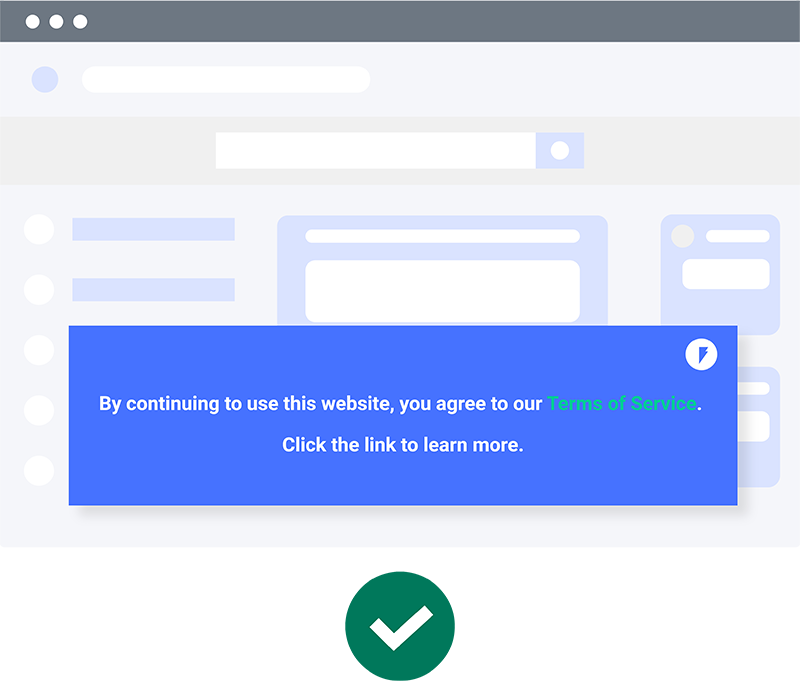Along the top of the image, there is a long gray bar stretching across the width. To the left of this bar are three small white circles. Below the gray bar, the background is a light gray with various elements in light blue. 

There is a light blue circle placed prominently towards the left. Next to this circle, there is a long horizontal oval. Below these elements, a white rectangle is positioned with a blue square on its right side, containing a white circle inside the square. 

Continuing with the light blue background, there are two long horizontal rectangles situated on the left side. 

In the center of the image, a blue rectangle measuring approximately five to six inches in length and about four inches in height takes focal attention. In the upper right corner of this rectangle, there is a white circle featuring a blue lightning bolt inside. 

Within the blue rectangle, white text reads: "By continuing to use this website, you agree to our terms of service." This text has a green accent. 

A prompt below encourages action with the text, "Click the link to learn more."

Located about three inches below the blue rectangle, there is a large green circle featuring a white checkmark inside. The large green circle with the white checkmark inside is repeated again about three inches further down.